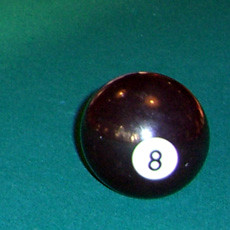The image is a small, square photograph featuring a close-up of an actual black billiard 8 ball, positioned towards the lower right-hand corner against what appears to be a green felt surface of a pool table. The green has a soft, almost teal hue, and the surface maintains a consistent depth of color, though it appears slightly lighter towards the upper left corner. The black 8 ball has a white circle with a black number 8 at its center, which is oriented towards the right side of the image. The ball reflects multiple lights from above, with a notably bright light just above the number 8 and several yellowish reflections near the top, likely from overhead fixtures. The reflections suggest a well-illuminated environment, potentially a bar or lounge.